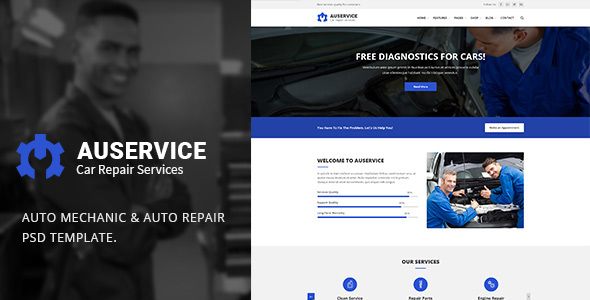This is the homepage of a business website for "AUSERVICE Car Repair Services Auto Mechanic and Auto Repair PSD Template." The left side of the webpage features a striking black-and-white image of a man standing in an auto repair shop. In the foreground, to the left center, there's a prominent icon of a wrench inside a bracket. On the right side of the page, a set of comprehensive menus with multiple drop-down options are available for easy navigation through the services provided by AUSERVICE.

Central to the layout is a colorful section displaying an image of a mechanic wearing blue work attire, likely protective clothing or a jumpsuit, as he inspects a car. This image is accompanied by a banner that highlights a special offer: "Free Diagnostics for Cars."

Below this banner, a welcoming message reads "Welcome to AUSERVICE," followed by a gray menu bar featuring a detailed list of available services, each represented within blue circular icons. Additionally, there is a contact section for visitors seeking further information.

Towards the top section, a series of symbols is displayed, along with a photograph of two mechanics in jumpsuits working on an engine. One mechanic gives a thumbs up with his left hand, while the other, a blonde man, smiles directly at the camera, adding a friendly and approachable touch to the website.